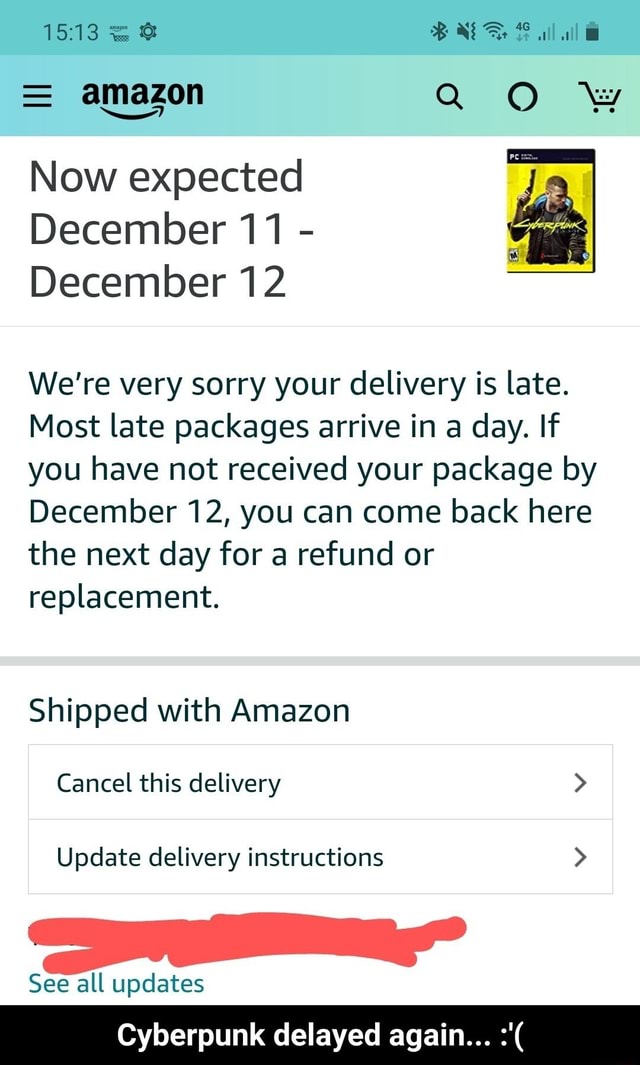The image is a screenshot of the Amazon website, captured on a mobile device. At the top of the screen, there is a greenish-blue header displaying the time "15:13" in dark gray text. In the upper right corner, there are icons indicating that Bluetooth is on, notifications are off, Wi-Fi is on, and the battery is nearly full.

Below the header, there's a light greenish-blue banner with the black Amazon logo on the left side and a shopping cart icon on the right. The main content area features a message against a white background with gray text, stating: "Now expected December 11th through 12th. We're very sorry your delivery is late. Most packages arrive in a day. If you have not received your package by December 12th you can come back here the next day for a refund or replacement."

A gray horizontal line separates this message from the subsequent text in black, which reads "Shipped with Amazon." Following this is a box containing options to "Cancel this delivery" with a right-facing arrow, and "Update delivery instructions."